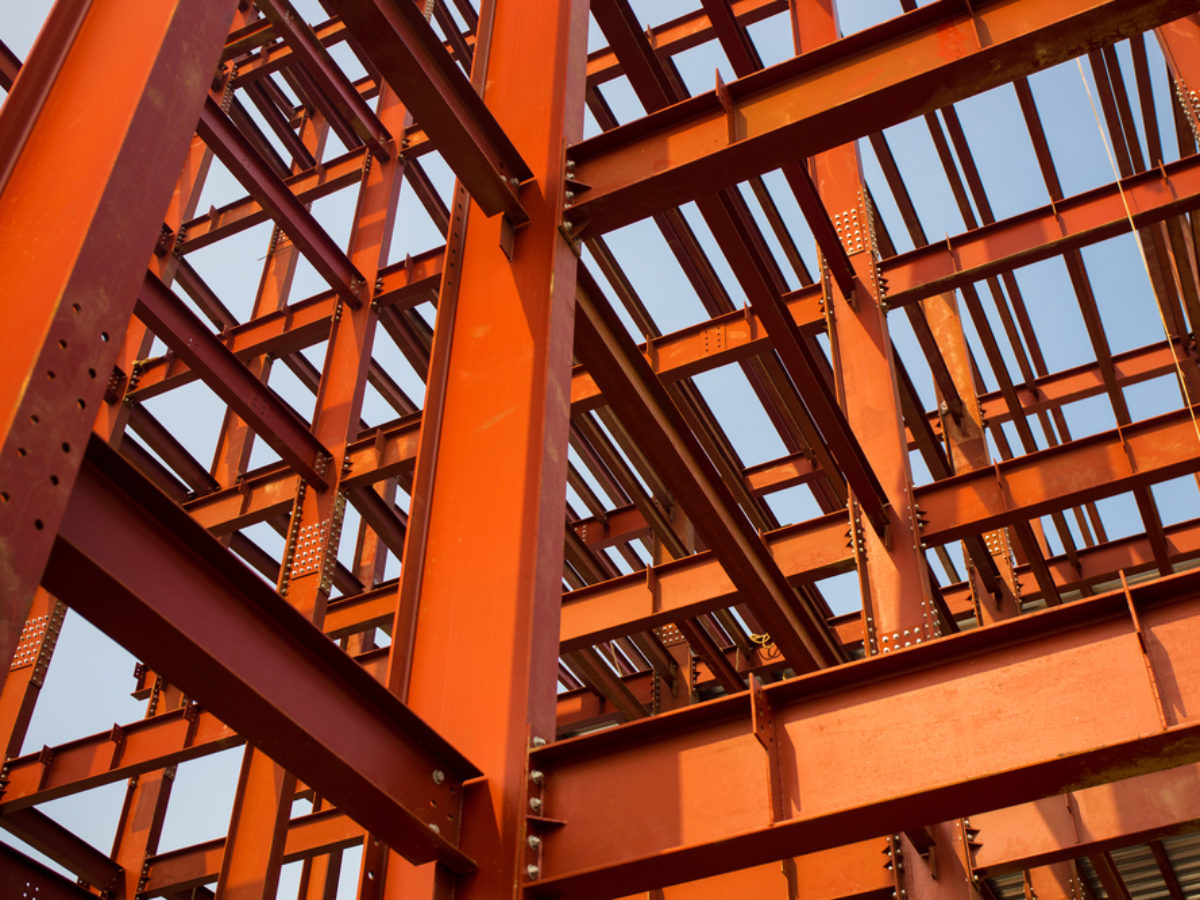The image reveals a dynamic construction scene, showcasing the early stages of a high-rise building or commercial property, defined by its striking steel framework. The vibrant structure, predominantly composed of crisscrossed I-beams, stands out in two distinct hues—vibrant orange and a dark reddish-orange. The photo is taken from the ground, looking up through the intricate web of beams, giving a sense of scale and complexity to the steel skeleton against a beautiful baby blue sky. The beams are new, shiny, and free of rust, adorned with numerous bolts and plates, evidencing their robustness and the modernity of the construction. The sizable upright beams, possibly measuring around 8 by 12 inches, alongside the substantial crossbeams, indicate a highly engineered structure built to support significant weight, poised to become a massive, resilient edifice once completed.